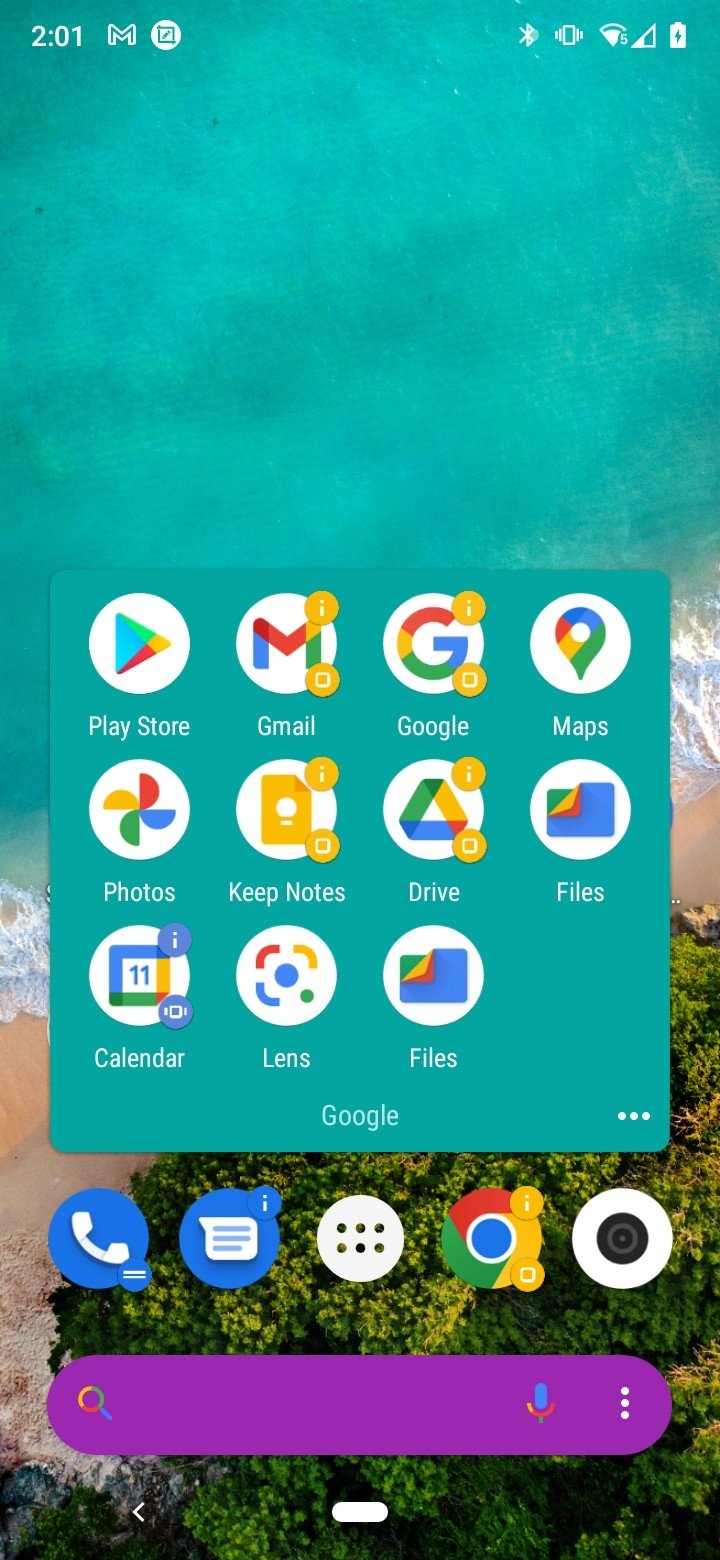Screenshot of a smartphone home screen displaying a battery percentage of 201% with a charging symbol. The background image features a picturesque beach scene with a tree. The screen is populated with various app icons including Play Store, Gmail, Google, Maps, Photos, Keep Notes, Drive, Files, Calendar, Lens, and Files again. At the bottom, there is the Google search bar, three horizontal dots indicating more options, and a row of five icons featuring a blue circle with a phone symbol, a hamburger menu, a chat symbol in a blue circle, an eye icon, an icon with six small circles (three on top and three below), the Google Chrome symbol, and a camera lens.